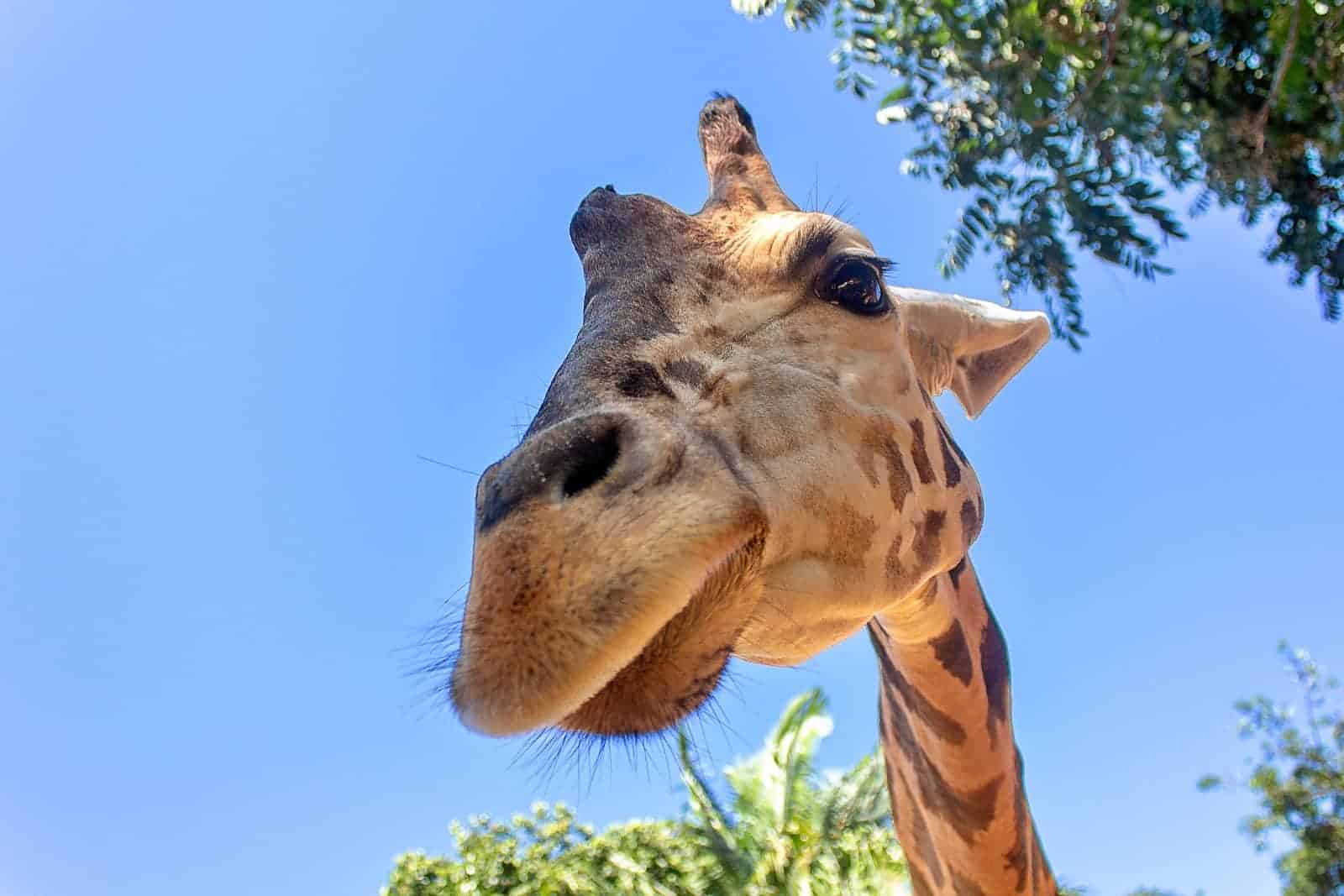This is a highly detailed, close-up, macro photograph of a giraffe, taken from a low angle looking up, which gives the impression that the giraffe is leaning down towards the camera. The focus is predominantly on the giraffe's face, with the nostrils and mouth being the largest and most prominent features. The viewer can see the giraffe's black nostrils, textured fur with light tan skin interspersed with dark brown patches, the large inquisitive eye, and even the fine black whiskers around its mouth. Notably, the giraffe's eyelashes are visible, adding to the intimate depiction. 

The photograph appears to be taken outdoors during the day, under a clear, light blue sky without a single cloud. The background includes out-of-focus green foliage, highlighting the foreground further. There are a few dark and light green leaves from nearby trees framing the edges of the image. No text or humans are present, giving full attention to the giraffe’s captivating expression as if it's curiously looking at the viewer, adding a sense of whimsy and engagement. The giraffe’s short horns and the ridge atop its nose are also distinguishable, along with parts of its long neck extending downwards and out of focus.